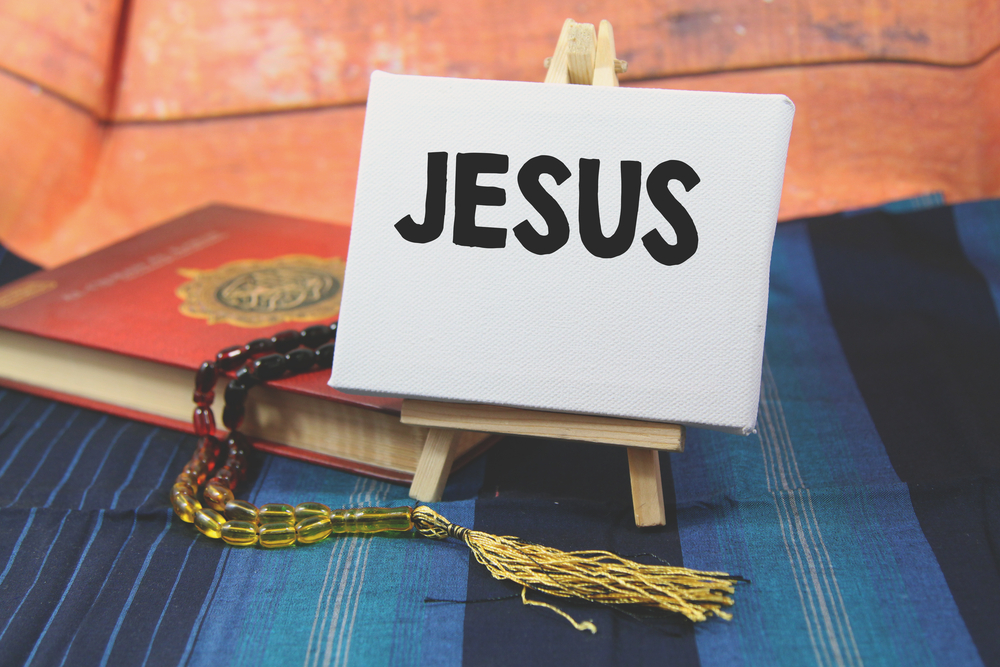In the foreground, positioned on a horizontally aligned, blue cloth with a mix of white, darker blue, and white lines, stands a small, unpainted wooden easel shaped like an "A". The easel holds a white board, displaying the word "JESUS" in bold, black, all-capital letters. Resting to the left of the easel is a hard-covered red book featuring a yellow emblem at its center. Draped over the book is a rosary composed of dark red and orange beads, complete with a yellow tassel. The backdrop of this scene is an orange wall, somewhat blurred at the top, giving an older, weathered appearance with hints of white and gray detailing. This detailed tableau captures a serene and reverent setting, combining elements of spirituality and simplicity.